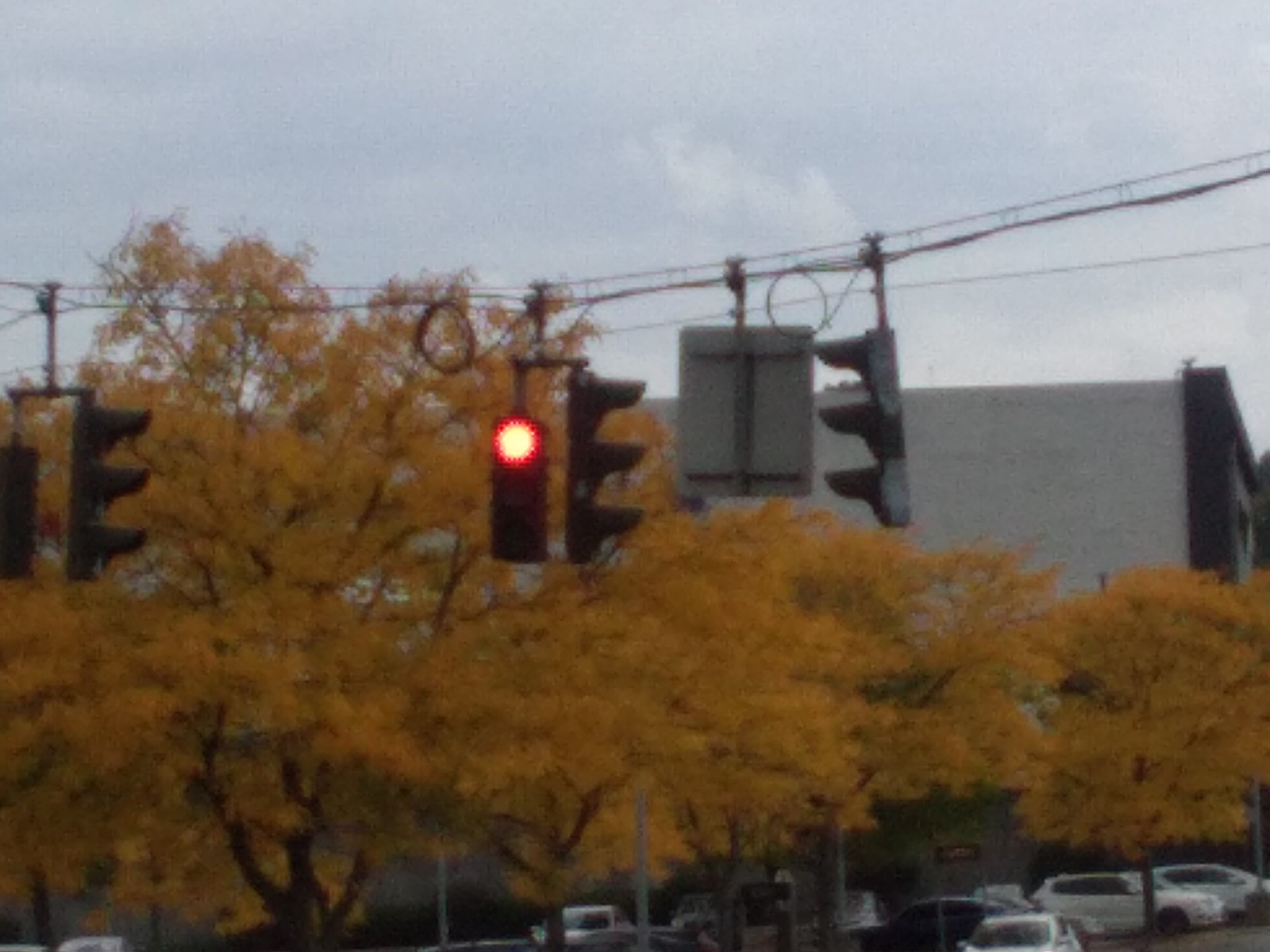The image depicts a cluster of five traffic lights suspended from a long black wire, with one light prominently displaying a red signal towards the camera while the others are angled towards the right and left. The scene is set against an overcast sky, lending a white, cloudy backdrop. Surrounding the intersection are several trees adorned with yellow and golden-brown leaves, indicating a seasonal shift. Nestled among these trees are multiple parked cars, predominantly white, with a black car also visible. Additionally, a sign whose message is obscured from view hangs between two of the traffic lights. The partial view of a white building is noticeable in the background, contributing to the urban setting of the photo.